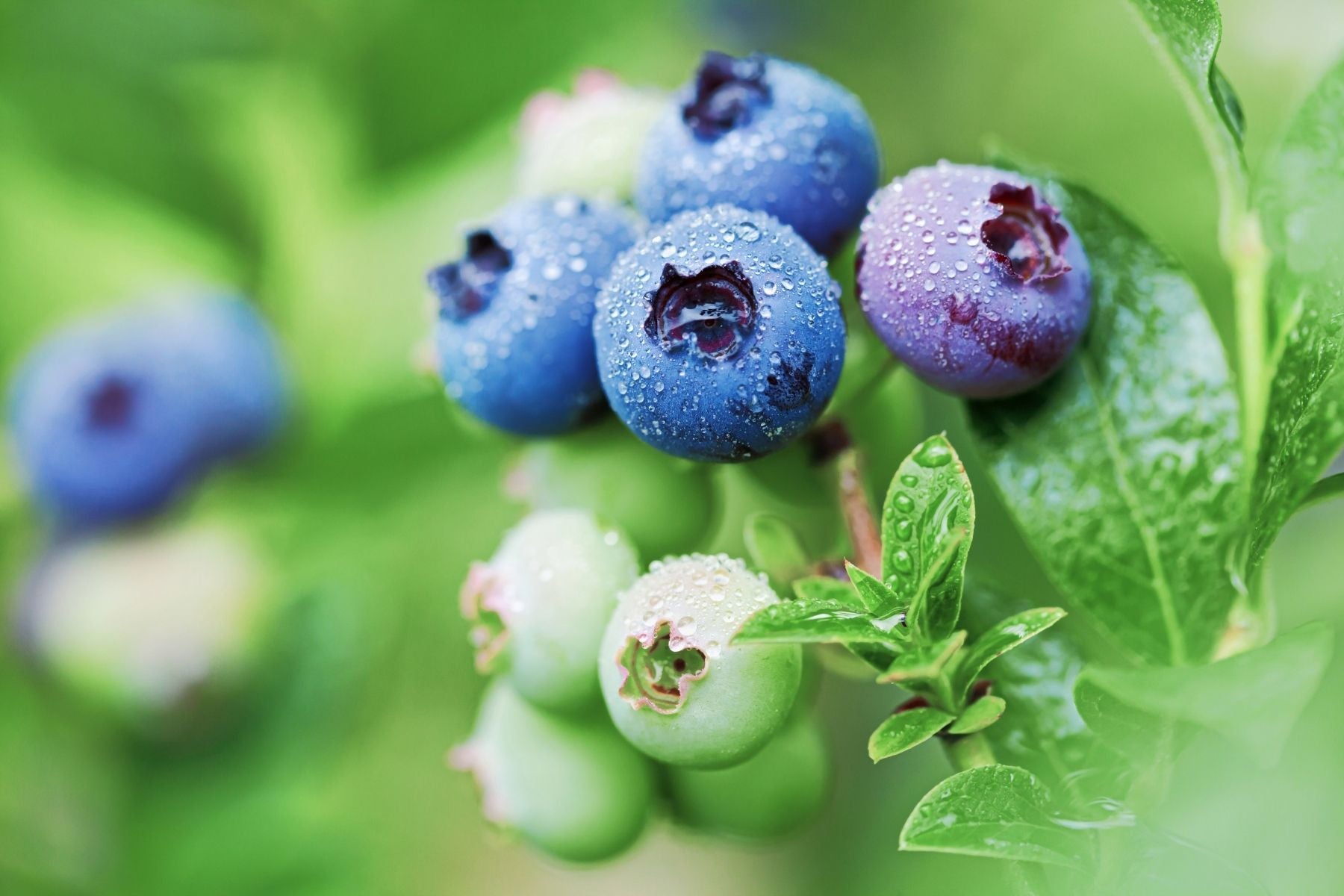This detailed close-up image captures a section of a blueberry bush with berries in different stages of ripeness. At the top of the image, there are four to five ripe, blue blueberries and one that is a rich purple. Below these, towards the bottom, are four green, unripe blueberries. Each blueberry prominently features a small central hole. The right foreground is in sharp focus, with vibrant leaves in good condition and visible water droplets, suggesting the photo was taken after a rain or in the morning dew. The background on the left side of the image is blurred, adding depth and highlighting the focused berries and leaves. The overall scene balances sharp, detailed elements with a softer, green-hued backdrop, emphasizing the natural beauty and vibrancy of the fruit and foliage.